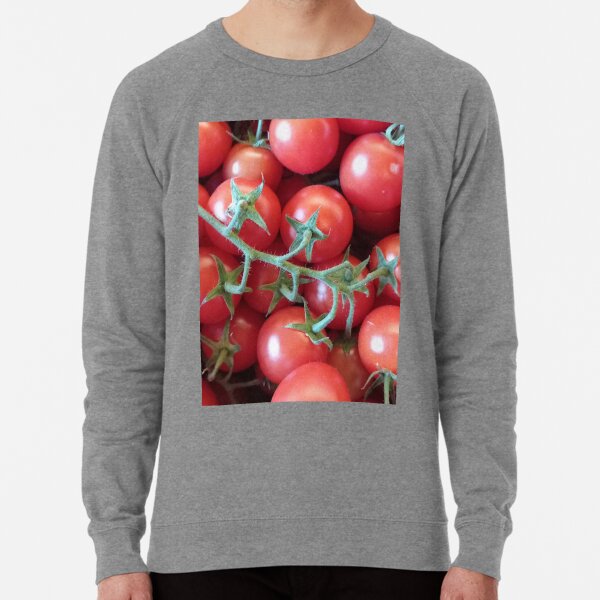This product image, likely from an online retail platform like Etsy or Amazon, features a Caucasian man with lightly tanned skin modeling a long-sleeved, heathered gray shirt. His facial features, save for a hint of stubble on his chin, are cropped out of the image. The background is entirely white, placing full emphasis on the shirt. The centerpiece of the shirt is a large, color photographic print of numerous red tomatoes attached to a green vine, complete with tiny prickly details. The tomatoes vary in visibility, with some fully visible and others partially obscured. The model's arms hang relaxed at his sides, and he is also wearing dark blue jeans or black pants.